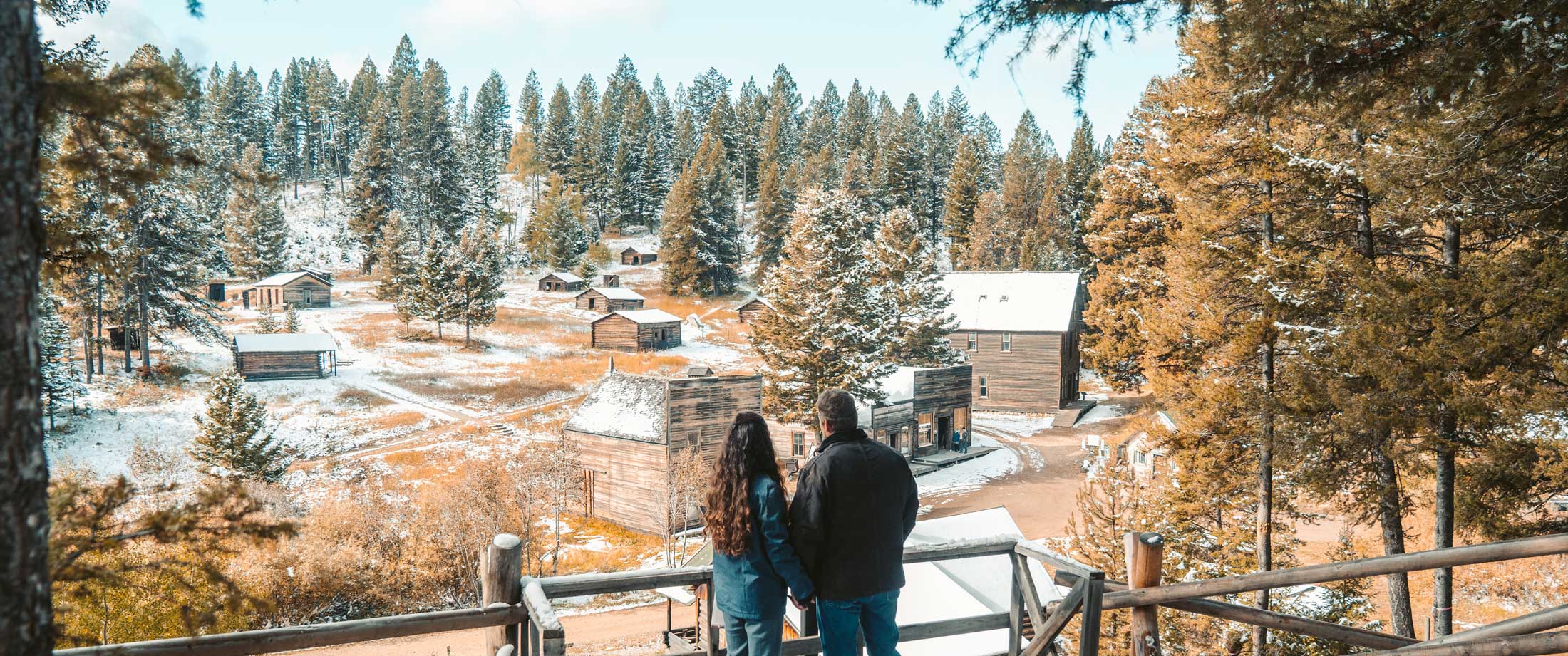This photograph captures a couple standing on a wooden balcony or descending stairs, looking out over a picturesque, snow-dusted frontier village nestled in a forested landscape. The scene is framed by tall evergreen pine trees, their branches sporadically sprinkled with snow, and patches of snow covering the ground, suggesting a setting in wintertime or early spring. 

The couple is intimately positioned, holding hands, with the woman dressed in a teal blue jacket and jeans, her long brown wavy hair cascading down her back. The man, with short gray hair, is also clad in a blue jacket and jeans. Below them, the rustic village unfolds, comprising an array of one-story wooden buildings and cabins scattered amidst the trees. 

At the center of their gaze are rows of wooden buildings, resembling an Old West downtown area with storefronts and possibly a bar, a barn, stables, and houses. The village is interconnected by one or two main roads or loops, edged up along a gentle hill. No other people are visible, leaving the couple alone to enjoy this serene vista.